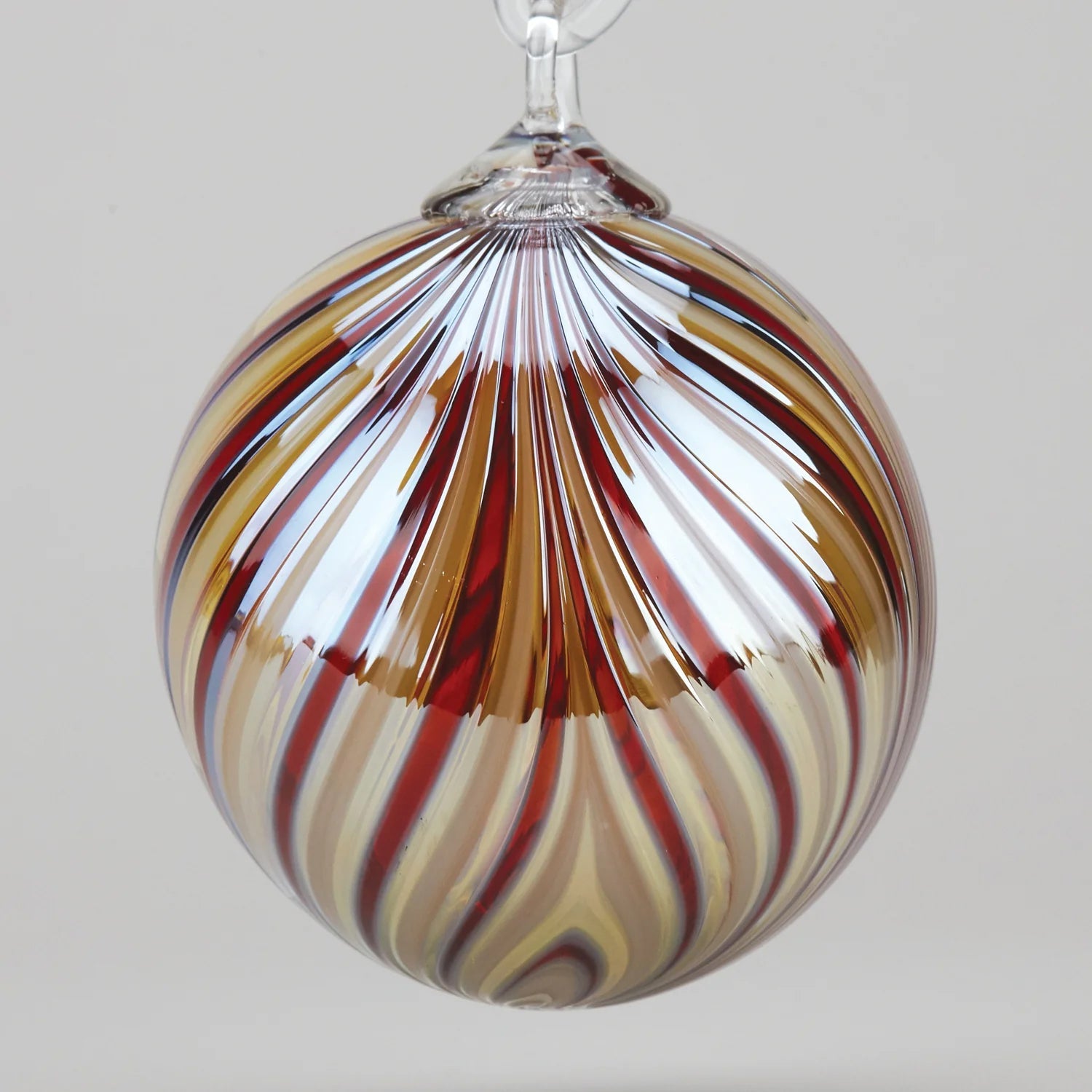This image showcases a stunning, spherical Christmas ornament made of blown glass. The ornament is attached to a clear, see-through blown glass hanger that loops up to a delicate chain, also resembling glass. The ornament's surface features intricate strands and stripes of vibrant colors, including reds, golds, and burgundies, along with varying shades of beige and opaque yellows. The darker brown coloration seems to be more pronounced halfway up the ornament, creating a striking contrast against the lighter colors. The ornament is well-lit, highlighting its shiny, glossy finish and making the rich colors pop against the plain white background. This elegant decoration hangs gracefully, drawing attention to its detailed craftsmanship and vivid hues.